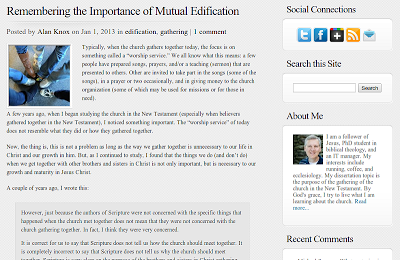This image is a screenshot of a blog post with a light gray background. The headline, located on the upper left, reads "Remembering the Importance of Mutual Edification" and indicates it was posted by Alan Knox on January 1st, 2013. Just below the headline and author's name is a small photograph showing the feet and lower legs of approximately four or five individuals, all wearing blue jeans and sneakers. 

The text of the article is in small, somewhat blurry font, making it difficult to read. In the upper right-hand corner, there is a section for social connections. This includes a white square containing icons for various sites: a blue 'Tumblr' icon, a blue Facebook icon with a white 'F', a black icon with a plus sign for additional options, an orange RSS feed icon with curved lines, and an email icon. Below these icons is a search box, followed by a brief bio of the author Alan Knox. Underneath the "About Me" headline, there is a headshot of the author, depicting a white man with graying hair who appears to be in his mid to late 50s. The bluriness of the font also obscures the reading of his bio.